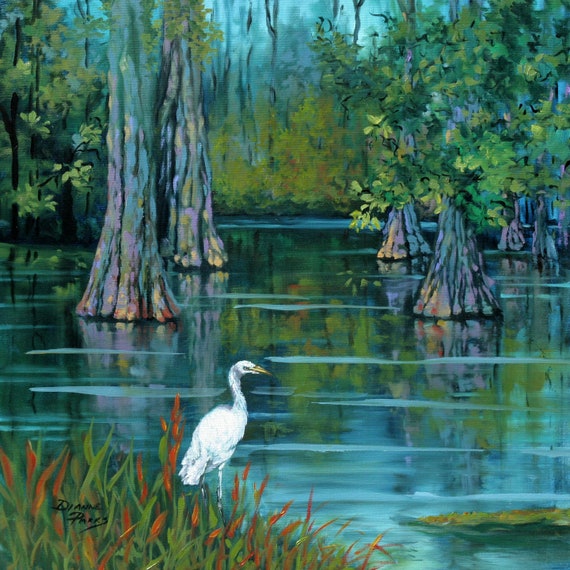This captivating painting, titled "Louisiana Swamp Painting with Egret and Bald Cypress Trees" by Dianne Parks, exquisitely captures a serene swamp scene. Dominating the center, a white egret with a yellow beak stands gracefully at the edge of calm, light blue water, seemingly on the lookout for fish. Tall green and brown grass, interspersed with striking orange blades, occupies the bottom left, where the artist's signature, "Dianne Parks," is visibly inscribed. The swamp, with its reflective still waters, is populated by several imposing cypress trees, their trunks emerging robustly from the water and capped with lush green leaves. These leaves and trunks cast gentle, mirrored reflections upon the water's surface. The background of the painting transitions into a light blue sky where the trees gradually fade, creating an ethereal atmosphere that enhances the tranquil beauty of the swamp.